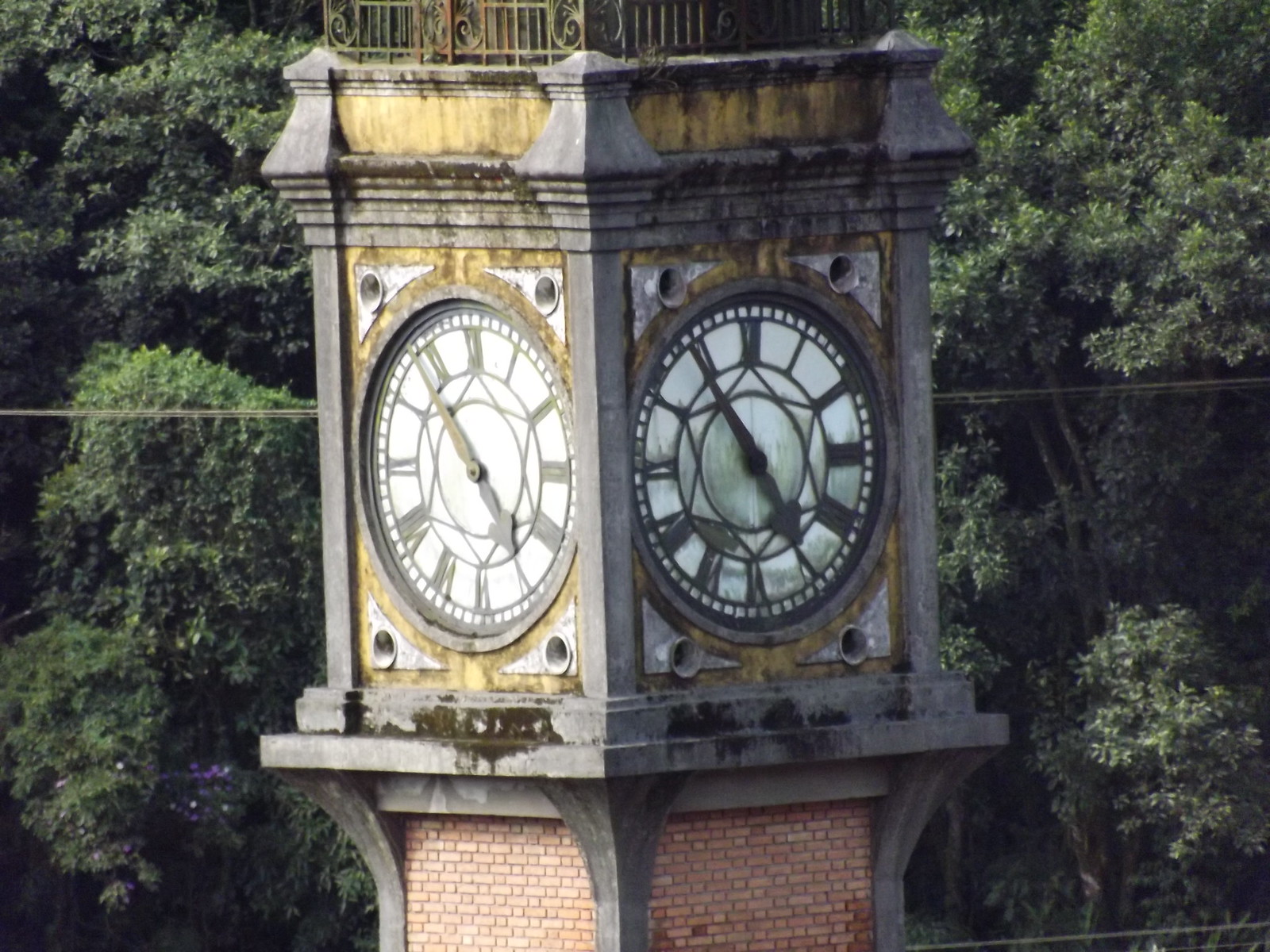A towering clock structure stands prominently against the backdrop of silhouetted trees and interspersed power lines. The clock, situated atop the tower, is visible on all four sides, with each circular face uniformly displaying the time, which appears to be around 3:54. The clock's face is a distinguished white, contrasted by its dark brown Roman numerals and hands, lending a vintage charm to the timepiece. The tower itself, tall and weather-worn, exhibits signs of age with patches of rust and dirt, hinting at a storied history.